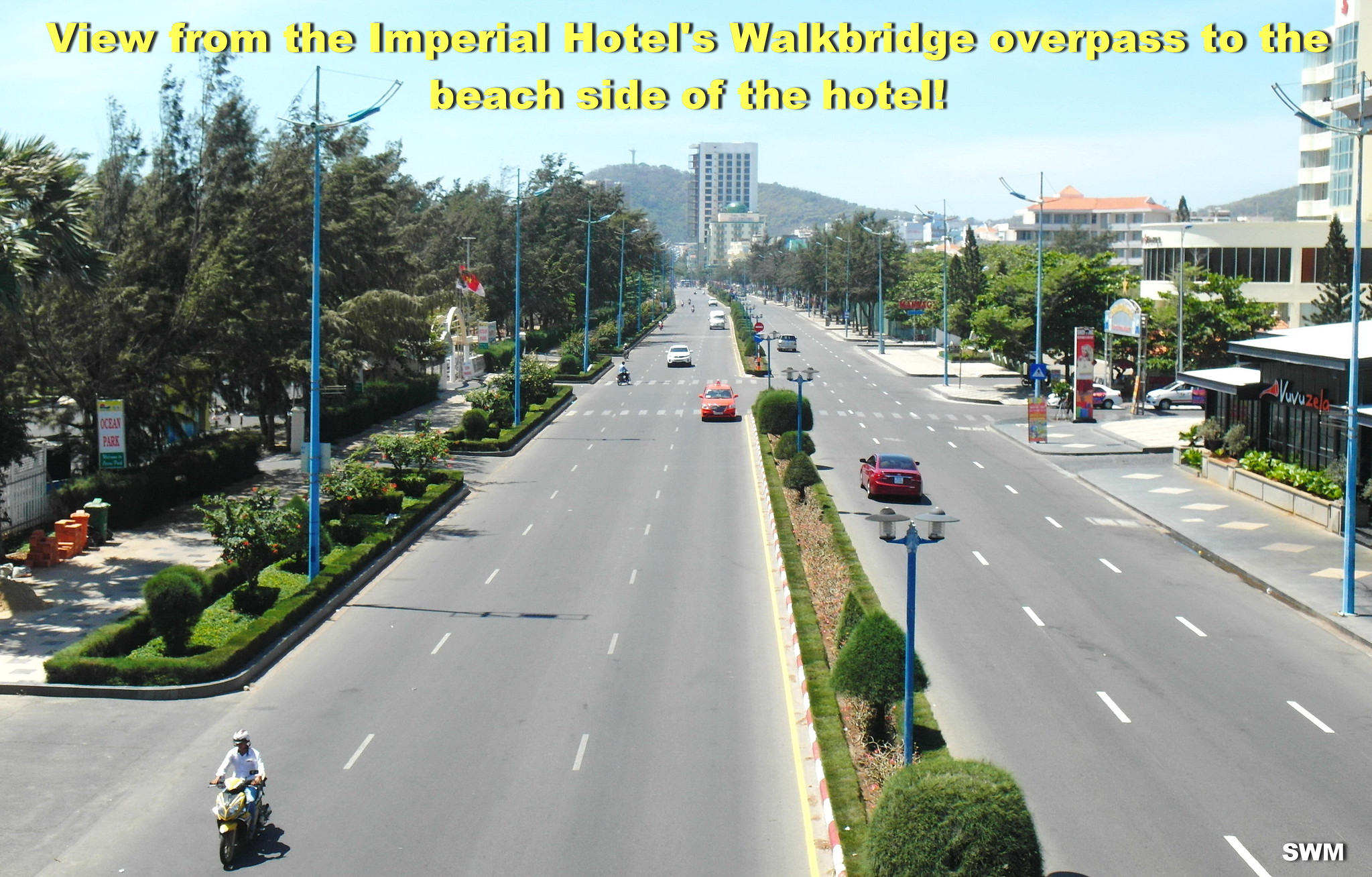This is a detailed photograph with yellow text at the top reading, "A view from the Imperial Hotel's walk bridge overpass to the beach side of the hotel." The image captures two adjacent streets, each flowing in opposite directions. The main road is notably large, featuring three lanes in each direction, making it a six-lane thoroughfare. The streets are flanked by buildings on both sides; the left side appears residential with well-landscaped green grass and bushes, while the right side has many stories and various structures, with tall blue streetlights lining the sidewalks. The center median separating the two streets is also meticulously landscaped with trimmed bushes and trees, contributing to the pristine appearance of the road. Sparse traffic includes cars and motorbikes, and there are no pedestrians visible on the sidewalks. In the distance, scattered skyscrapers emerge against a light blue sky, with hills and additional buildings forming the backdrop. A red flag with a yellow star on the left side of the street suggests the photograph was taken in Vietnam. The overall impression is one of an orderly, well-maintained urban area, possibly featured on a postcard due to its clarity and composition.